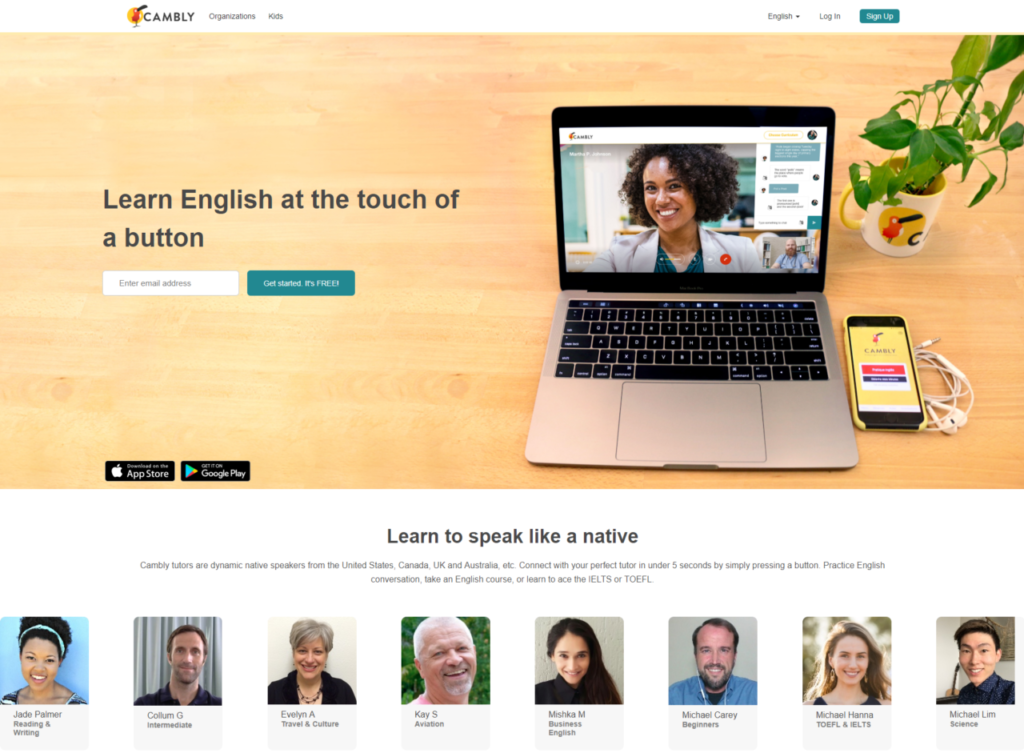The image showcases the homepage of the Cambly language learning website, set against a predominantly white background. At the very top of the page, the Cambly logo is prominently displayed on the left, followed by navigation links including "Organizations" and "Kids." On the right-hand side, there are options to select the language for the page, currently set to English, as well as "Login" and "Signup" buttons, with the "Signup" button highlighted in a greenish color.

The centerpiece of the layout is a stylized banner depicting a wooden desk. To the right on the desk, a laptop is shown with the Cambly website open, accompanied by a smartphone displaying the Cambly app and a pair of headphones. A small plant in a mug adds a touch of greenery behind these items. To the left of this setup, the text "Learn English at the touch of a button" is prominently displayed above an email entry box and a greenish "Get Started – It's Free" button. The lower left corner includes buttons to download the app from the App Store and Google Play.

Beneath this banner, set against a white background, a heading reads "Learn to speak like a native," followed by smaller text: "Cambly tutors are dynamic native speakers from the United States, Canada, UK, and Australia, etc. Connect with your perfect tutor in under five seconds by simply pressing a button, practice English conversation, take an English course or learn to ace the IELTS or TOEFL." Below this description, an image displays eight tutors, highlighting the variety of specializations they offer, from TOEFL and IELTS preparation to reading and writing, catering to beginners, intermediate, and advanced learners alike.